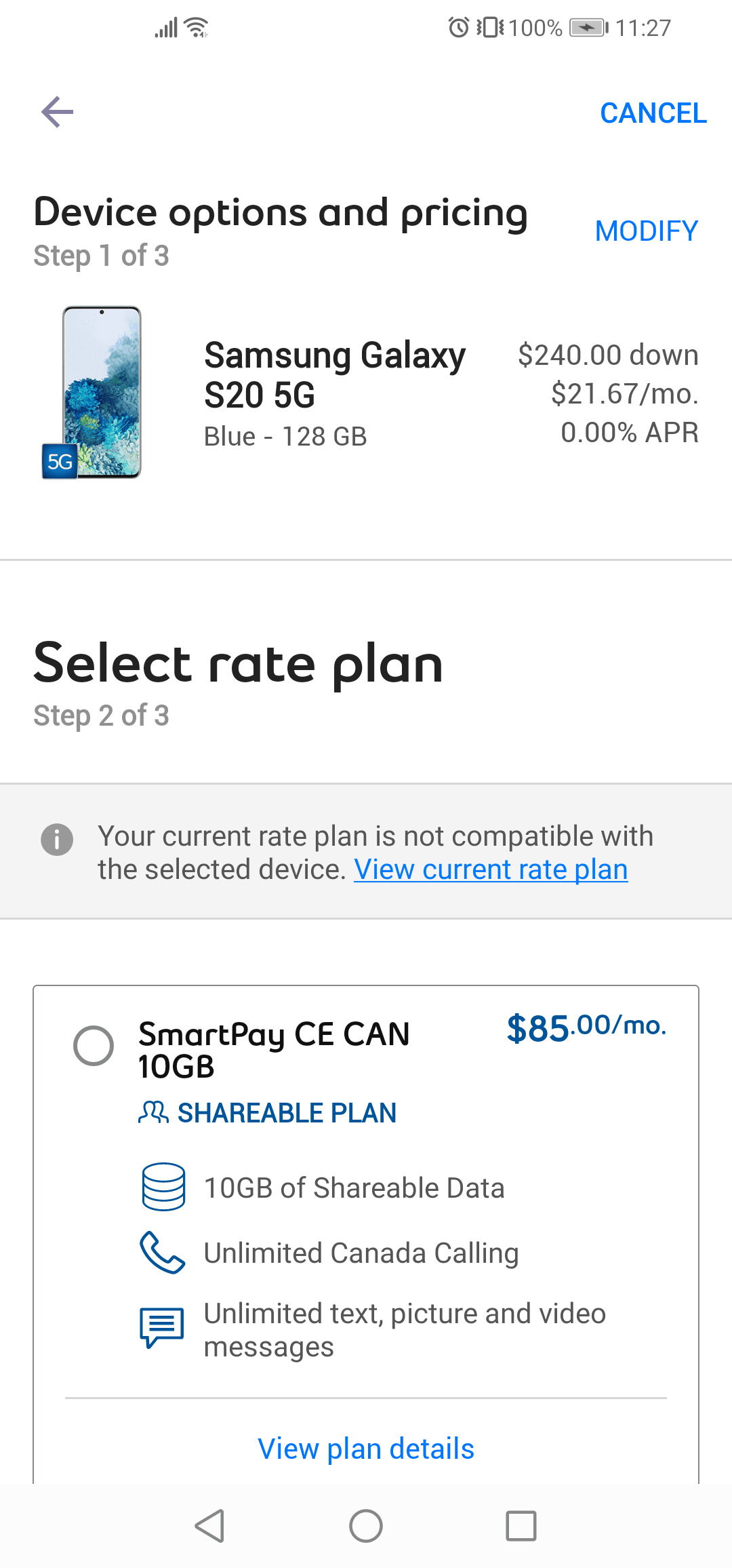This image is a cell phone screenshot that provides detailed information about a cell phone plan. The screenshot itself is taller than it is wide and features a white background, making it appear seamless and blending into the prolific space. 

In the upper-left corner of the screenshot, there is no carrier information visible, but signal strength and Wi-Fi icons are present. In the upper right corner, there are several icons, including an alarm clock, a symbol indicating the phone is set to vibrate, a battery icon showing 100% charge, and the time displayed as 11:27. There is also a blue "Cancel" button in the upper right corner and a back arrow in the upper left corner.

Below these indicators, the text "Device options and pricing, step one of three" is displayed. The screenshot reveals that the person is in the process of purchasing a Samsung Galaxy S25G in blue, with 128 gigabytes of storage. The financial details for the phone show a down payment of $240, monthly payments of $21.67, and 0% APR.

Further down, "Step two of three: select rate plan" is indicated. A highlighted box informs the user that their current rate plan is not compatible with the selected device and offers the option to view the current rate plan. Below this, there is one available choice for the new plan, displayed within a box with a radio button: the "SmartPay CECAN 10-gigabyte shareable plan" priced at $85 per month.